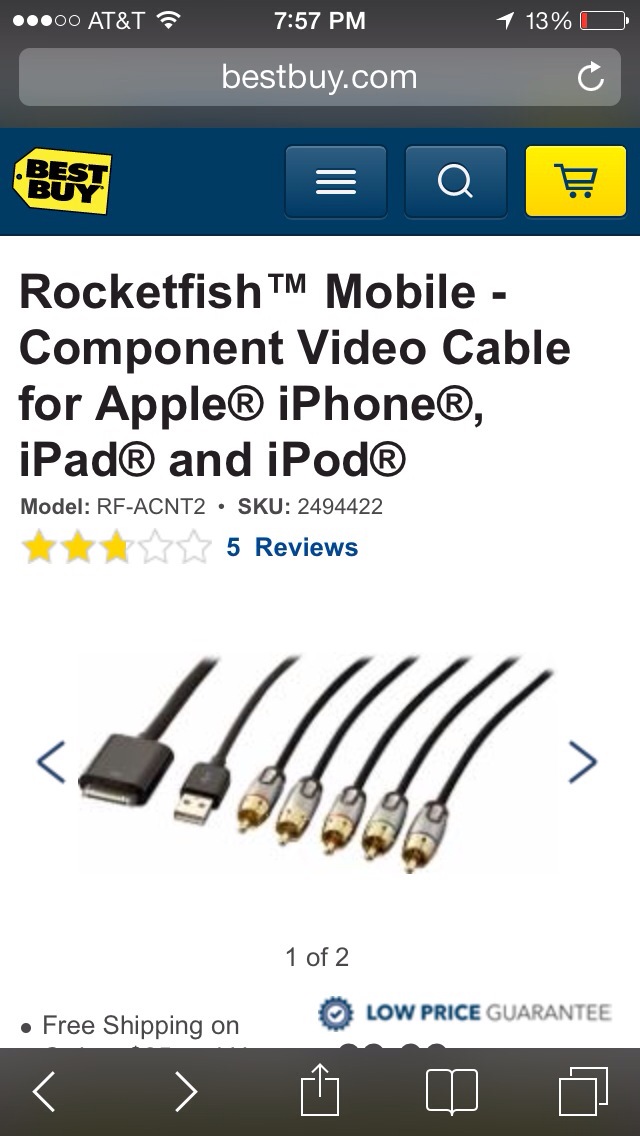The image is a tall, rectangular screenshot from a phone displaying a Best Buy webpage for Rocketfish Mobile Component Video Cables compatible with Apple iPhone, iPad, and iPod. At the top of the screenshot, the phone details are visible with "AT&T," the time "7:57 PM," and a battery level of "13%." Below that, the Best Buy website is labeled with a gray header showing "bestbuy.com" and a yellow tag-shaped logo with "Best Buy" in blue capital letters on a dark blue rectangle. The product listing includes the text "Rocketfish™ Mobile Component Video Cable for Apple, iPhone, iPad, and iPod" along with the model number "RFACNT2 SKU 2494422." The item has five reviews, averaging about three out of five stars, depicted with three yellow stars. The image predominantly shows the tips of various cables, including a USB cable and additional ports. The bottom of the screenshot mentions "free shipping" and "low price guarantee," though parts of these phrases are cut off. The overall screenshot captures the user's screen activity while browsing the Best Buy website at 7:57 PM with 13% battery remaining.